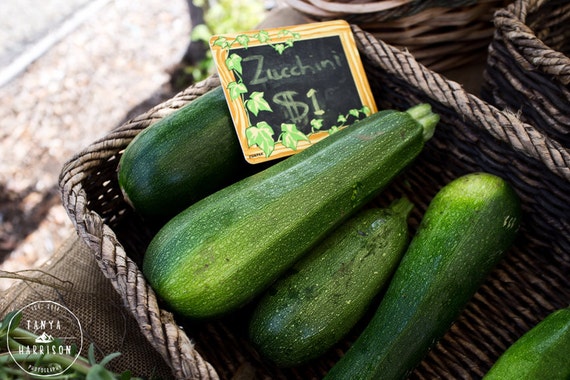This detailed close-up photograph showcases a dark brown wicker basket filled with an assortment of zucchinis of varying sizes and shapes. Some zucchinis are long and skinny, while others are wider and taper off. The zucchinis display a deep green color with light green splotches and a few scars, indicating their freshness. Inside the basket, resting on a burlap cushion, is a small wooden-framed chalkboard sign with green leaf embroidery around the edges. On the black chalkboard, written in green chalk, is the text "Zucchini $1." To the left of the main basket is another green vegetable, partially cut off in the frame, and there are two additional wicker baskets visible in the background on the right. The image is taken during the daytime, with the edge of the sidewalk and a piece of the road faintly visible on the left. The photograph bears a watermark in the bottom left corner, which reads "Fenya Harrison" with a circular mountain icon in between the name.